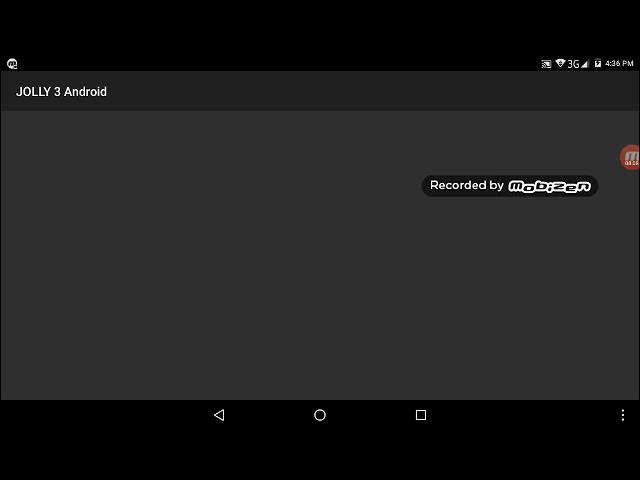A detailed descriptive caption for the image provided:

"This image portrays a square layout with distinct sections. At the very top, a long black bar spans the width of the image. On the lower left side of this bar, there is a circular white symbol featuring a black 'M' inside, whose significance is unclear. To the far right of the same bar, familiar smartphone symbols are displayed: a Wi-Fi icon facing a filled square, a downwards pointing arrowhead symbol, a 3G indicator with four out of five bars highlighted in white, and a padlock icon. Additionally, there is a white box with a black lightning bolt, possibly indicating charging status, and the current time displayed as 4:36 PM.

Below this black bar is a long gray bar with the word 'JOLLY' in all caps followed by the number 3 and the text 'Android cat;' the 'A' in 'Android' is lowercase. The central portion of the image is dominated by a large light gray box. Towards the upper right corner of this box, an oval-shaped black box contains the text 'Recorded by Mobizen' in white outlined letters with a blue accent, presented in a futuristic font.

Adjacent to this text, towards the upper right, is a partially visible orange or red circle with a lowercase 'm' inside and the number 326 beneath it. The circle is slightly cut off at the edge. At the very bottom of the image, another long black bar features a play button, a circle, and a square, all in white with black centers. Finally, on the far right of this bottom bar, three white dots are vertically aligned."